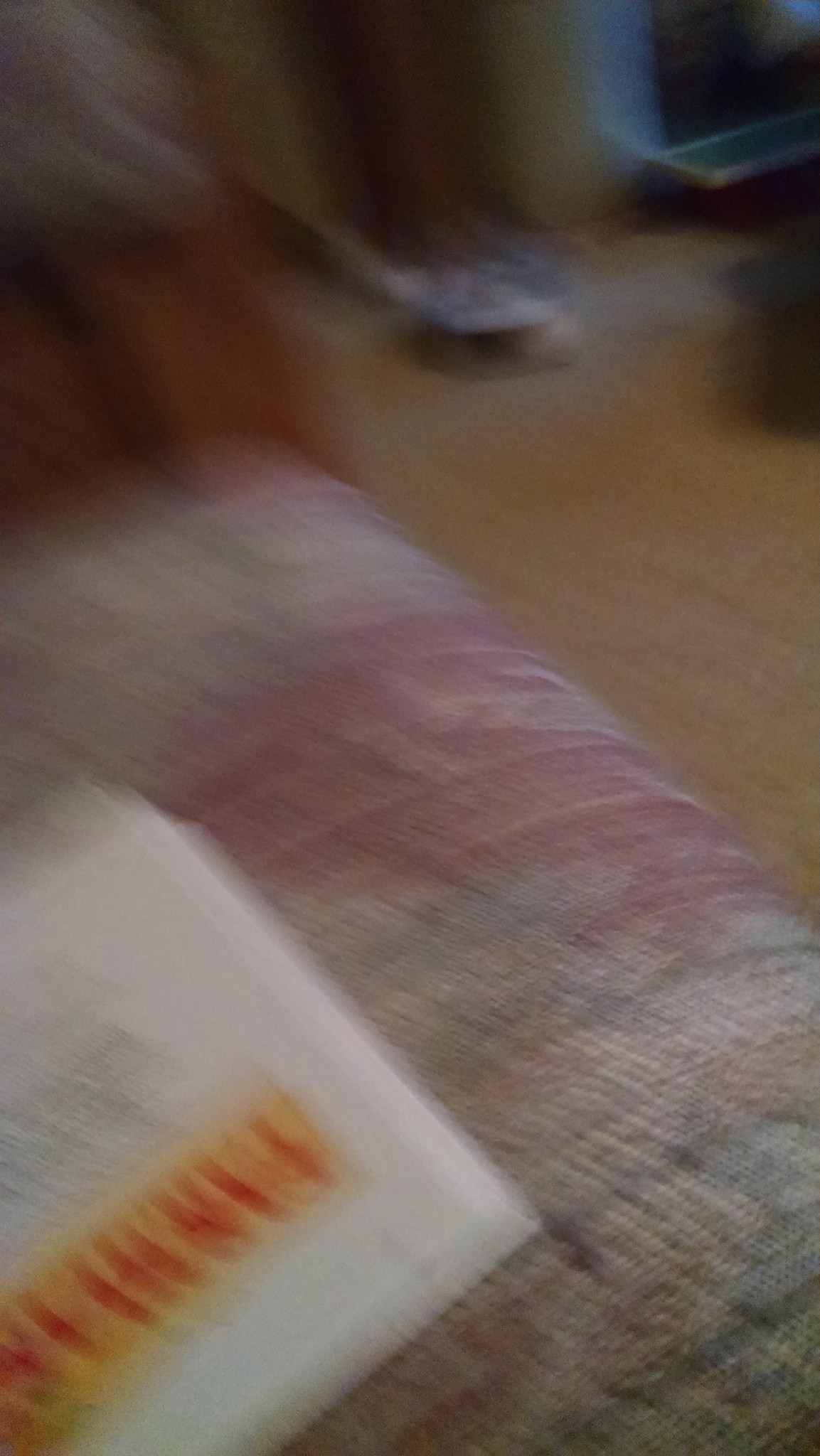This is a highly blurry color photograph of a living room setting. In the forefront, the edge of a multi-colored fabric couch appears, blending shades of red, white, and green, possibly with a wooden frame and armrests on the left side. Papers lie on the couch, marked by a large yellow rectangle with prominent red text and additional black text passages. Toward the bottom of the image, there's a textured cloth surface with pink, grey, and blue weaving. In the bottom left corner, there's a small square white object featuring indistinct red and yellow print with smaller black writing beneath. The possible blurry outline of a person is slightly visible, holding something that might be a vacuum cleaner or a vague whitish object on the ground. The surrounding floor is brown, and in the top left corner, a blue object with a lighter blue stripe and a dark blue shelf is discernible.